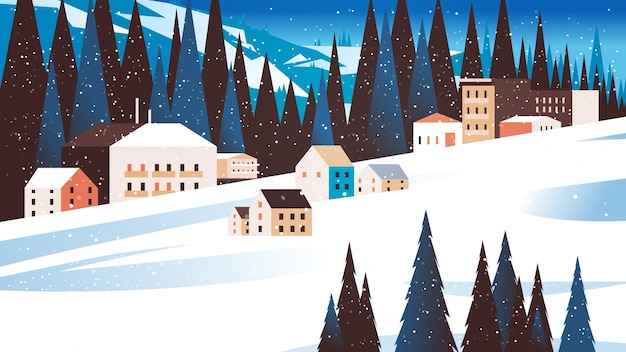The image is a detailed, stylized scene resembling a Christmas card or a 3D picture of a peaceful, sleepy snowy village. Dominated by a striking contrast of bright and dark blues, black, white, peach, orange, and gray, the scene is set against a backdrop of gentle snow-capped mountains and a brilliant blue sky. Snow falls softly from above, blanketing the landscape. In the foreground, various buildings of different shapes and colors—ranging from white with an orange front to blue and three-storied with a brownish-orange facade—dot the snow-covered ground. Interspersed among the buildings are an array of Christmas trees, depicted as upside-down triangles in deep blues and blacks, casting elongated shadows on the snow. The distinctive color palette and serene composition evoke a tranquil, wintry atmosphere.